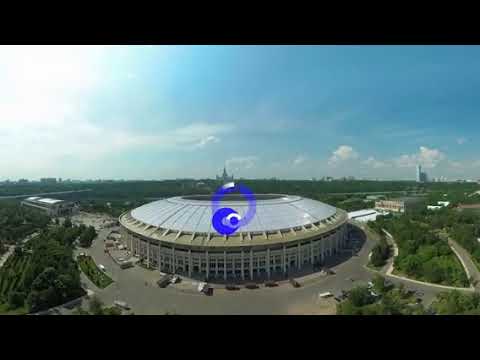This detailed photograph, taken from a high vantage point on a bright, sunny day, captures a large, circular, dome-shaped stadium prominently positioned in the center. The dome's rooftop is silver, bordered by a distinctive blue ring, with an additional softer blue ring atop it. The structure is surrounded by a gray pavement or street. A few cars are parked sporadically around the building, but the area seems mostly devoid of traffic. The scene is framed by lush, green trees and bushes encircling the stadium, extending out to a broader landscape dotted with more greenery, roads, and smaller buildings. In the distant horizon, faint outlines of taller buildings can be seen. The sky overhead is a brilliant blue, speckled with a few fluffy white clouds, bathing the entire scene in bright daylight. Notably, there is a blue watermark or symbol on top of the dome, suggesting a possible digital enhancement.